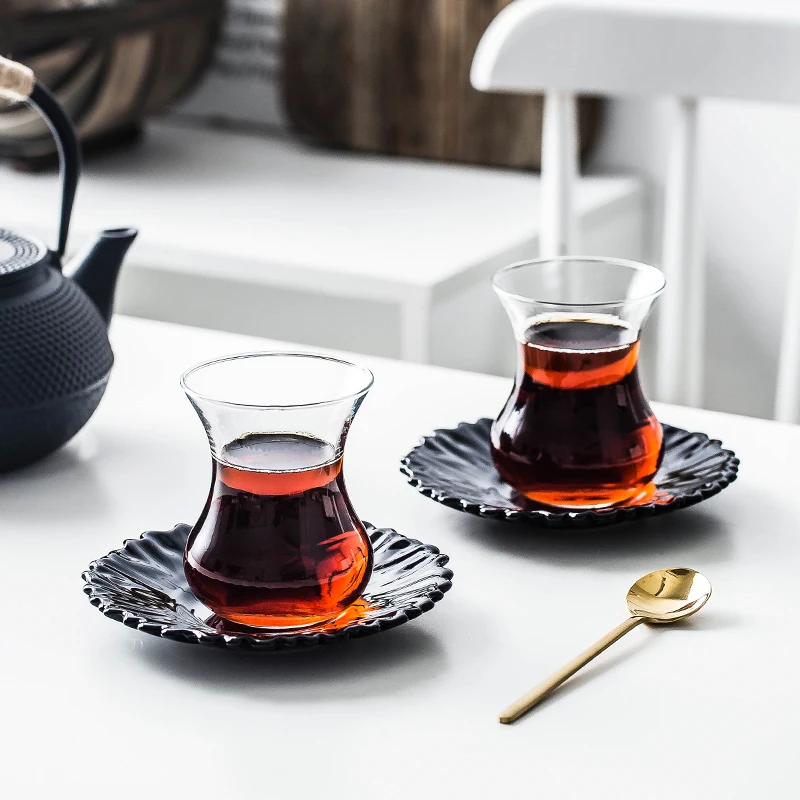The color photograph captures a detailed table setting on a white table, featuring two clear glass teacups filled three-quarters with a golden brown tea. The teacups have a unique shape, resembling flared Turkish teacups, with a narrowed neck and rounded bottom. Each teacup rests on a black, fluted-edge saucer. To the left of the image sits a dark gray cast iron teapot adorned with distinctive horizontal stripes and a beige-wrapped handle. A gold, round-tipped spoon lies near the saucers on the right side of the table. The background showcases a white wooden chair with a rounded top and vertical spindles, partially cut off on the right side, and a blurry second white table with assorted items, adding depth to the scene.